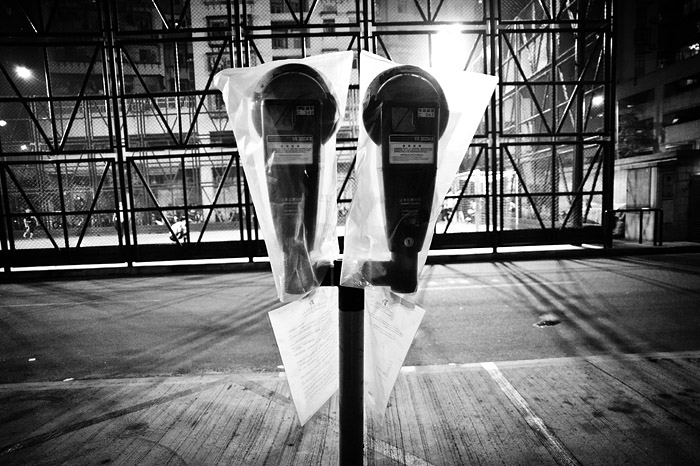This black and white photograph features a pair of parking meters located prominently at the center. Each meter is covered with a white plastic bag, from which a paper sign dangles, though the text on these signs is too small to discern. The meters stand on a walkway, possibly wooden with visible striations, that transitions into a conventional asphalt road to the sides and beyond. Behind the parking meters is a construction site filled with scaffolding and metallic structures, characterized by large, square frames of metal poles and diagonal supports, forming a dense, grid-like pattern resembling a soundstage or an enclosure. Further in the background, an apartment complex and what seems to be a stadium are visible, distinguished by a chain-link fence enclosing it and faint figures that could be considered players, especially on the left side. The scene is illuminated by very bright lights, suggesting the photograph was taken at night. The high contrast of the image makes the various elements—parking meters, scaffolding, and buildings—stand out starkly against the dark night backdrop.